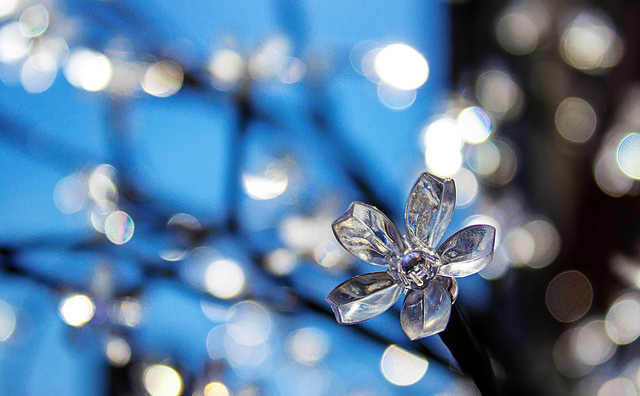This color photograph presents a stylized, intricate crystal flower, emerging from the bottom right of the frame. The flower, distinguished by its six translucent, semi-precious crystal petals, is the primary focus and is detailed sharply against a blurred background. The delicate flower is perched on a black stem, likely made of plastic. Surrounding the flower is a hazy backdrop, predominantly baby blue with sporadic black areas. The background features indistinct round circles of light—some translucent, others with a yellowish glow—giving an impression of water droplets or possibly additional stylized flowers. Thin dark lines, resembling branches or wires, crisscross the background, further accentuating the flower's clarity.